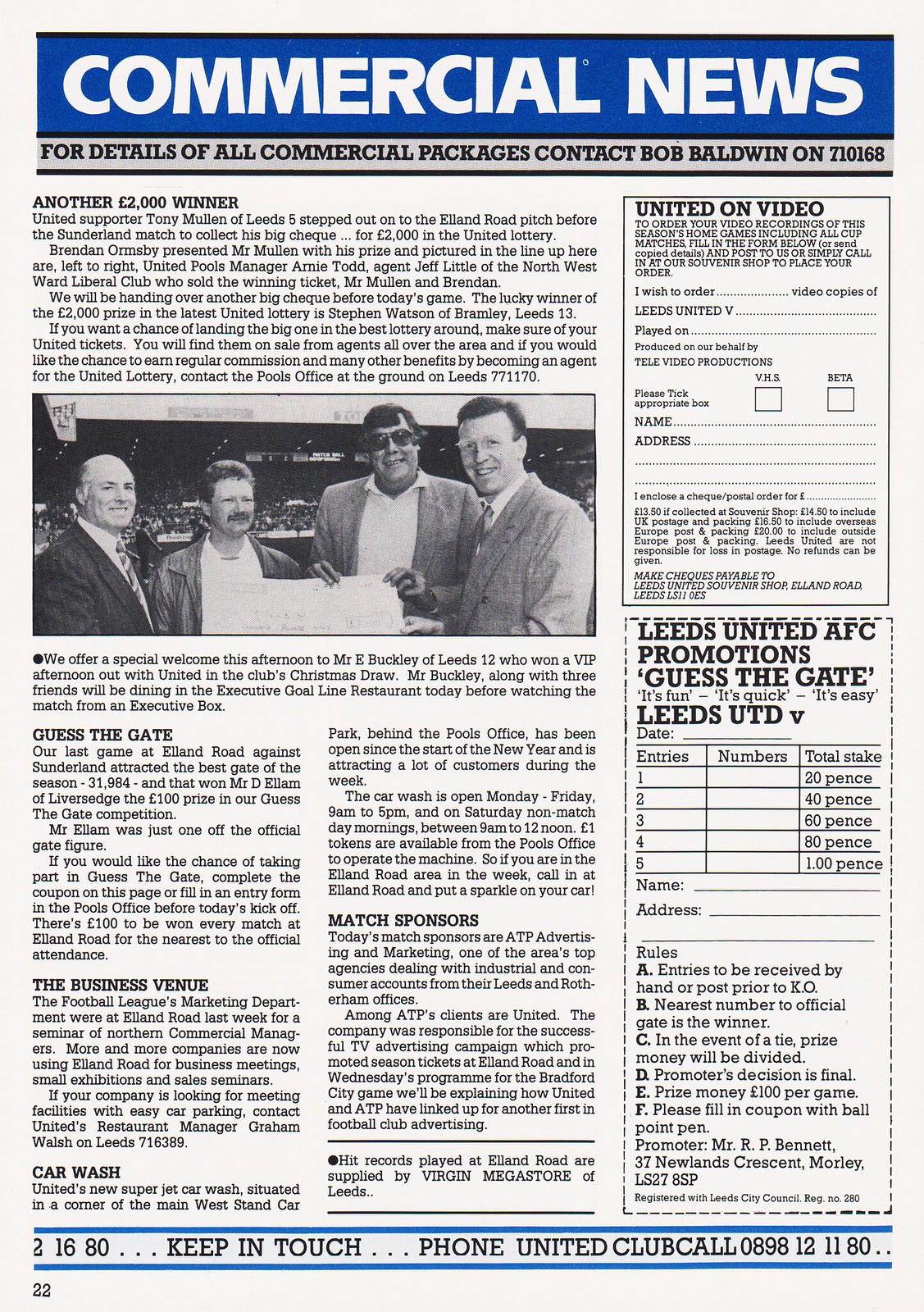The image shows a page, possibly ripped from a magazine or a newspaper, with a variety of details. Primarily black and white, it features a prominent blue headline at the top with white capital letters reading "Commercial News." Beneath this headline, there's a grey banner with black text that states, "For details of all commercial packages contact Bob Baldwin on 710168." 

The page contains a lengthy article section, under the title "Another $2,000 Winner," discussing various winners and other related topics in several paragraphs titled, "Guess the Gate," "The Business Venue," "Car Wash," and "Match Sponsors." Centrally, there's a slightly blurred black-and-white photograph of four men with dark hair, standing close together, one of them holding a large check in what appears to be a stadium setting.

In the left-center but more towards the top, the number 22 is printed in the bottom left-hand corner with a white border. The right-hand side features cut-out sections labeled "United Video," where readers can order video copies of the news program, and a Leeds United AFC Promotions Guess the Gate entry form. Finally, the bottom of the page has a blue banner with the text "Keep in touch. Phone United Club Call 0898-121180."